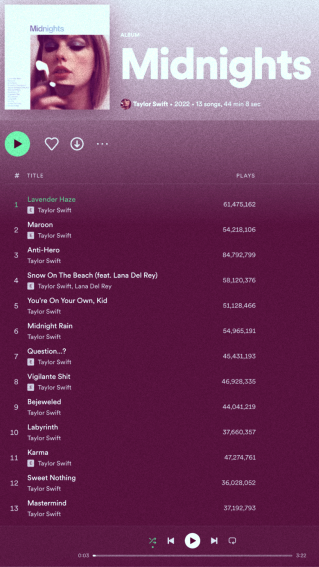This is an image depicting a webpage for Taylor Swift's album "Midnights." The top of the page prominently displays the album title, "Midnights," likely indicating it as the cover artwork or main title header. The page also specifies details about the album, including Taylor Swift as the artist, the release year of 2022, and the album's length—13 songs totaling 44 minutes and 8 seconds.

The interface highlights an active listening feature, with the song "Lavender Haze" indicated by a green font, suggesting it is either currently playing or available for playback by clicking a green circle with a play arrow. The page includes icons such as a heart, likely for favoriting tracks, and a download option for offline listening.

The full tracklist is visible, though somewhat difficult to read, listing songs as follows: "Lavender Haze," "Maroon," "Anti-Hero," "Snow on the Beach," "You're on Your Own, Kid," "Midnight Rain," "Question...?," "Vigilante Shit," "Bejeweled," "Labyrinth," "Karma," "Sweet Nothing," and "Mastermind."

The background color of the page is maroon, which complements the overall theme of the album. The bottom section includes a white circle with an arrow pointing to the right, possibly indicating navigation to the next page or additional options.